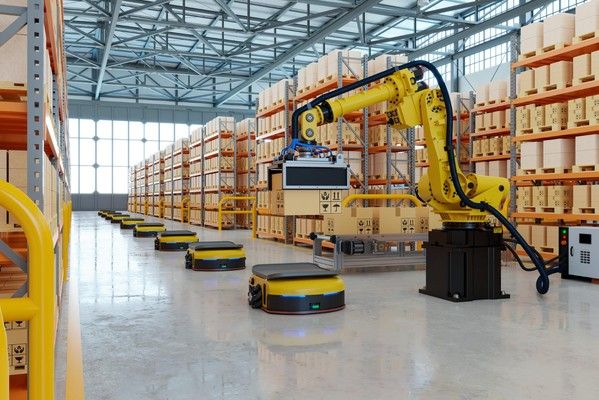The high-quality image showcases the interior of a large warehouse or manufacturing plant with a sophisticated setup. Central to the image is a bright yellow robotic claw machine poised on a dark black base. This articulating robotic arm is seen holding a beige box, appearing to lift it from or place it onto a black platform, possibly on a smaller robot equipped with small wheels and a flat top. The warehouse boasts high, metal, and coral-colored shelves stocked with numerous beige boxes. These shelves extend upwards almost reaching the ceiling, which is an intricate metal grid structure that also features opaque glass panels allowing a view of the sky. The warehouse floor is made of sleek, shiny material, likely gray marble. Additionally, there's a backdrop with metal poles and windows on the left, enhancing the expansive and industrial ambiance of the setting.